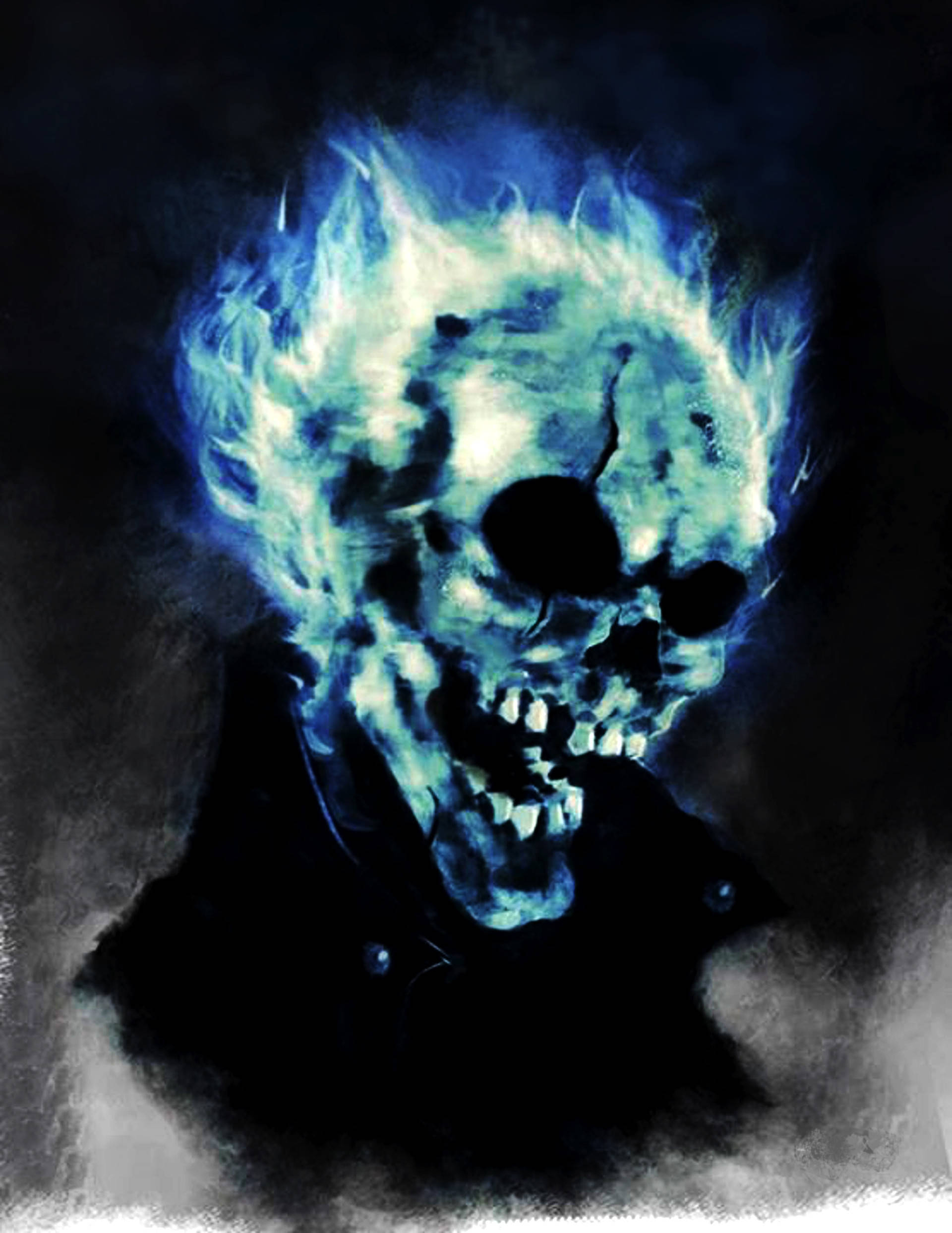The digital artwork features a human skull engulfed in vibrant blue flames, reminiscent of propane fire, with hues ranging from bright to dark blue. The skull, centrally positioned, seems to emit flames from its ears, cheeks, and the top of its head, creating a blur effect. Its eyes and nose are depicted as hollow black voids, while the mouth is wide open, revealing sharp, white teeth in a sinister, almost cynical laugh or scream. The lower part of the skull transitions into a dark silhouette, resembling a neck and collar area, surrounded by a lighter gray background that contrasts against the dark black hues. The background shifts from a deep black at the top to a gray gradient towards the bottom, enhancing the eerie and intense atmosphere of the print.